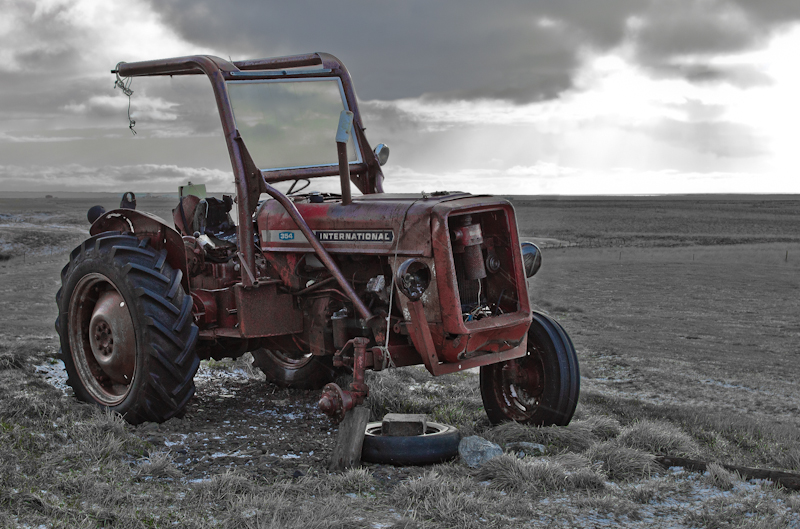This photograph features an antique, broken-down tractor prominently displayed in a barren field under a stormy sky. The image employs selective coloring, highlighting the faded, rusty red of the tractor against a primarily black and white background. The dark, heavy clouds above add a dramatic contrast, with a sliver of sunshine breaking through on the top right. The foreground shows an open field with very light, almost white grass, characteristic of a prairie landscape.

The tractor, identified as an "International," shows clear signs of abandonment and wear. It is supported by two large rear wheels with deep grooves for traction, and two small front wheels, though the front right tire is missing and the vehicle is precariously propped up by a wooden block. The detached tire lies flat on the ground nearby. The front right headlight is damaged, and the absence of a full seating area further underscores the machine's dilapidated state. The image captures the essence of decay and nostalgia, making it suitable as an artistic photograph for decor or display.